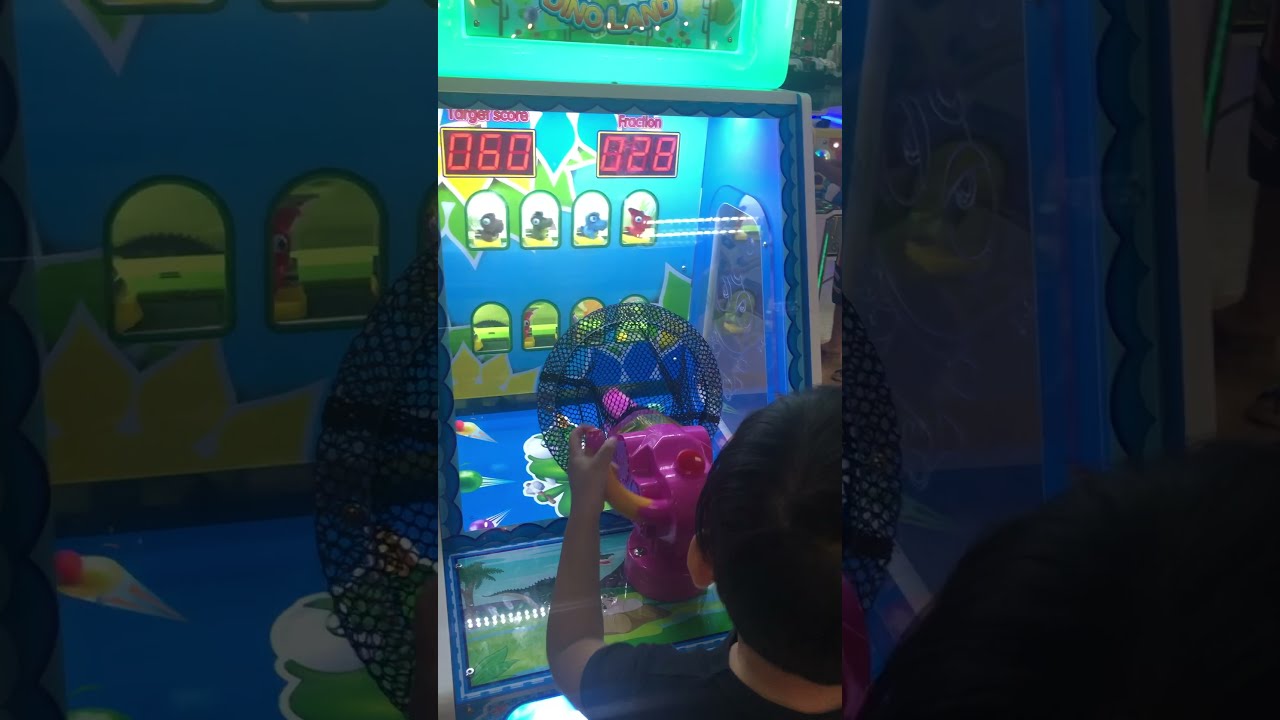In this arcade image, a young boy with short black hair, wearing a blue t-shirt, is intensely focused on an interactive shooting game. He is wielding a predominantly pink water gun with a yellow handle, equipped with what appears to be a see-through black ring at the tip. The game's display shows two red LED screens at the top; the left screen indicates the target score of 60, while the right screen shows his current score of 28. The game's screen is divided into sections, each containing various targets. The upper row consists of four differently colored alligators—black, green, blue, and red. The bottom row features four green cars. Below the rows, there is a cartoon drawing of an alligator with small bird-like figures pointing towards it. The backdrop of the game screen has a blue wall with rectangular openings that have rounded tops, adding to the whimsical setup. The overall scene evokes the lively atmosphere of an entertainment venue like Chuck E. Cheese, with the child deeply engaged in trying to hit his targets and improve his score.